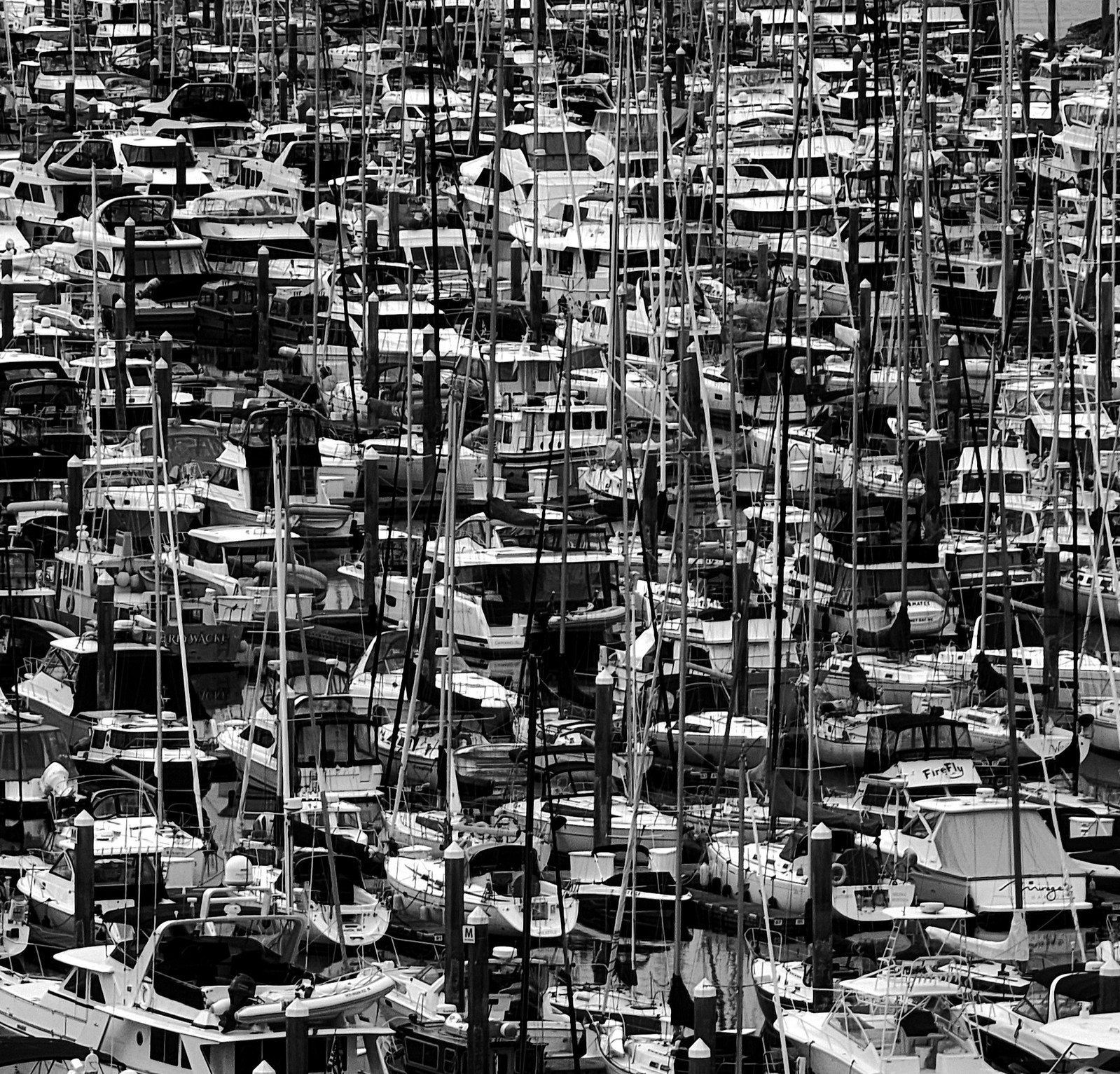This black and white photograph showcases an exceptionally crowded marina, densely packed with a staggering array of boats. The image captures various types of boats, including sailboats, cruisers, and commercial fishing boats, all crammed together to the point where the water is scarcely visible. The low angle of the shot accentuates the thicket of masts and poles rising from the boats, creating a chaotic and almost impenetrable scene reminiscent of a bustling junkyard rather than a serene marina. The boats span the entire frame, from edge to edge, with some labeled parking spots visible among the congestion, such as one marked with the letter "M". This captivatingly chaotic scene highlights the sheer volume and diversity of boats, making it one of the most packed marinas imaginable.